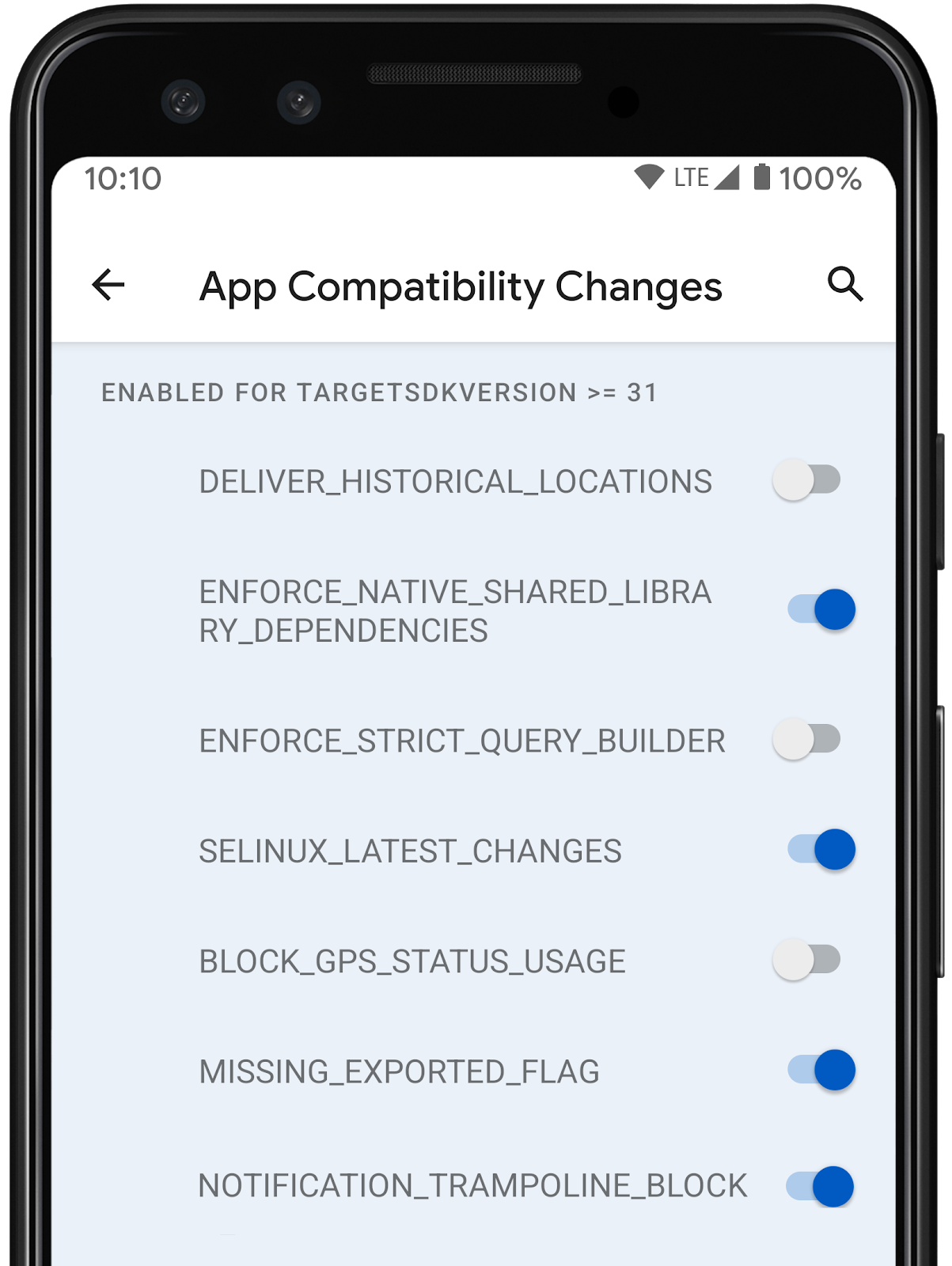The image displays a screenshot of a smartphone interface, likely on an Android or iPhone device, possibly a Samsung or iPhone. The upper portion of the screen is a white banner showing various status indicators: the time reads 10:10, LTE service is full, the battery is fully charged, and the Wi-Fi reception is strong. In black font within this white banner, the text "App Compatibility Changes" is displayed next to a magnifying glass icon for searching.

The lower section of the screenshot is grayed out. On the left side, in all caps and gray font, the text "ENABLED FOR TARGET SDK VERSION >= 31" is prominently displayed. Below this header, several settings are listed with their statuses:

1. **DELIVER_HISTORICAL_LOCATIONS**: Turned off
2. **ENFORCE_NATIVE_SHARED_LIBRARY_DEPENDENCIES**: Turned on
3. **ENFORCE_STRICT_QUERY_BUILDER**: Turned off
4. **SE_LINUX_LATEST_CHANGES**: Turned on
5. **BLOCK_GPS_STATUS_CHANGES**: Turned off

Overall, the image provides a detailed view of various app compatibility settings and their current states on the device.